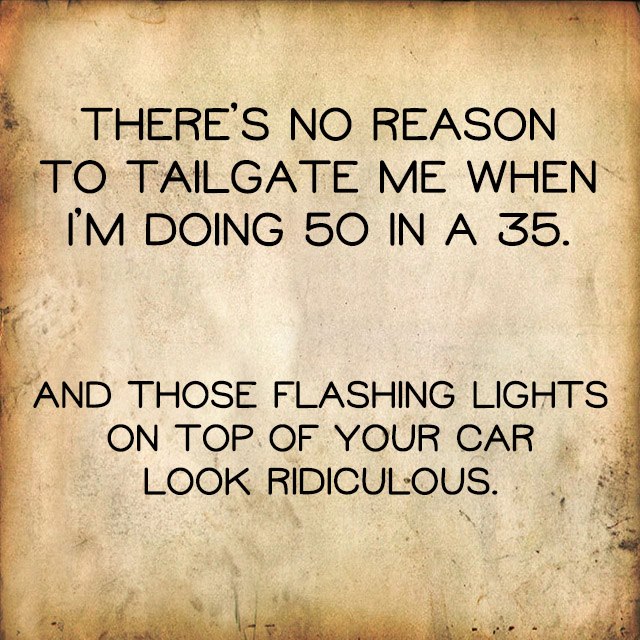This image, often shared on social media, features a humorous text designed to look like an aged, yellowing piece of paper with a light brown, almost stucco-like background that darkens towards the edges, giving it an old, vintage appearance. The text is centrally positioned and split into two sections, each consisting of three lines in a clear, black font. The upper section reads, "There's no reason to tailgate me when I'm doing 50 in a 35." The lower section humorously adds, "And those flashing lights on top of your car look ridiculous." The lettering is in all capitals except for the "I's," and there's a notable space between the two sections, emphasizing the joke about not realizing one is being pulled over by a police car and perceiving the situation as mere tailgating. The image, likely created using Photoshop, is a witty comment on misunderstanding police pursuits and is a popular type of post on platforms like Facebook.